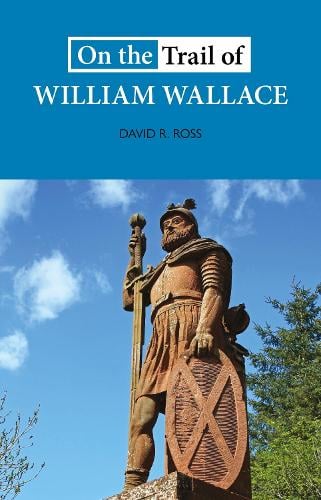The book cover for "On the Trail of William Wallace" by David R. Ross features a simplistic design primarily dominated by the title, which occupies about one-third of the image. The text, "On the Trail of William Wallace," is set against a blue backdrop, with different parts of the text rendered in white and black. The upper section of the cover includes a blue band, while the lower section transitions into an actual picture showcasing a sky with fluffy white clouds and green tree branches on the sides. Below the title is an aged statue, presumably of William Wallace, clad in a historically inspired armor ensemble that includes a kilt-like garment extending to his knees. The statue, which appears weathered and possibly rusted, depicts Wallace with a helmet, beard, and a shield marked with a giant X in one hand, and a sword in the other, posed as if in mid-action. The detailed attire and armament fittingly point to him being a notable Scottish warrior.